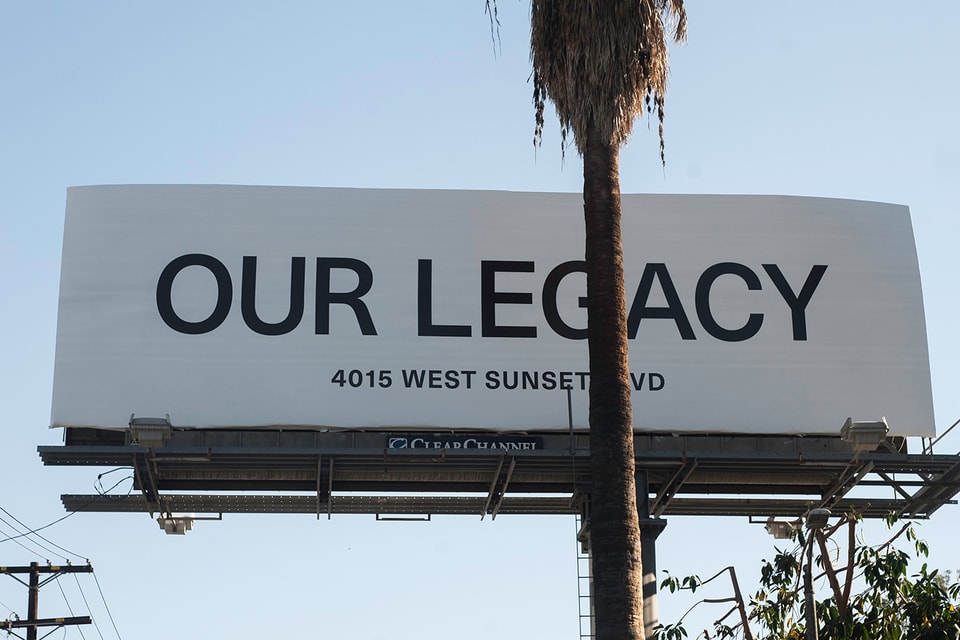The image depicts a large, white, plain-looking billboard with a prominent slogan "Our Legacy" in extremely large black capital letters. Below the slogan, in smaller text, it reads "4015 West Sunset Boulevard," and at the very bottom, it says "Clear Channel" in small print. The billboard is situated on a metal and wood platform equipped with a ladder for maintenance access. Dominating the scene, a very tall and thin palm tree with a narrow trunk stands right in front of the billboard, partially obscuring the letter "G" in "Legacy." The palm tree's fronds appear dry and dead. On the lower left corner of the picture, there are barely visible power lines stemming from a power pole. In the lower right corner, a smaller, green-leaved deciduous tree and some vegetation are visible. The sky is light blue with no clouds, suggesting a bright, clear day in a warm weather area. The image appears to be taken from the ground, capturing the street-side view with a backdrop of the clear, light blue sky.